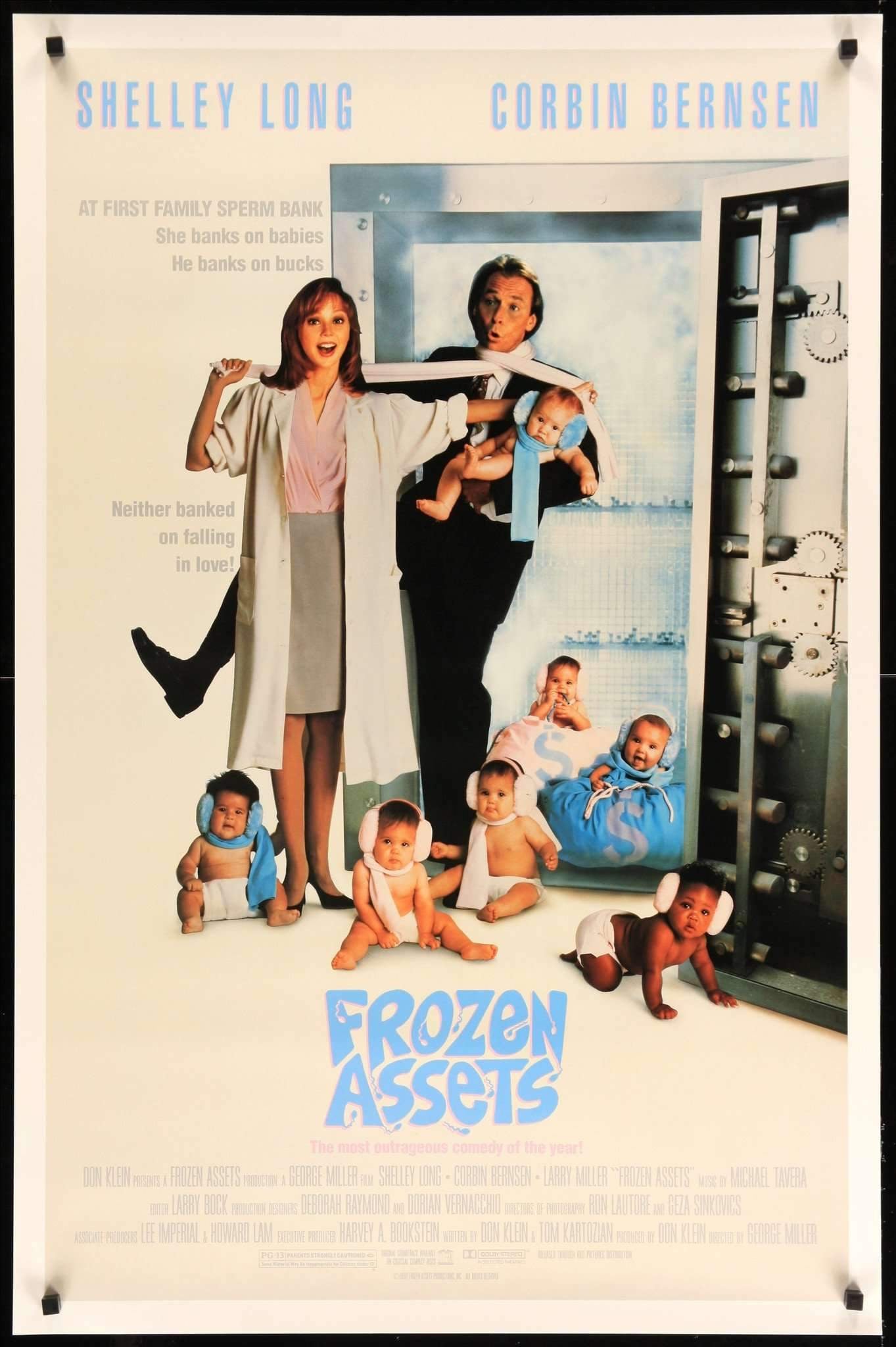The movie poster for "Frozen Assets" features a lightly weathered, off-white background framed by a black and white border, suggestive of an old, vintage look. The poster is securely attached at the corners, possibly with pins or clasps, to a vertical rectangle background. Prominently displayed in blue text at the top of the poster is the cast: Shelley Long on the left and Corbin Bernsen on the right.

In the central image, Shelley Long and Corbin Bernsen stand in front of what appears to be a vault or freezer. Shelley is dressed in a light-colored coat and playfully holds a scarf wrapped around Corbin's neck, who is attired in a black suit jacket with one leg humorously lifted. He cradles a baby in his arms, looking as surprised as Shelley.

Scattered around them are seven babies, four on the floor and two inside the vault, with another one crawling near the vault door. Notably, two babies are inside money bags, emphasizing the comedic and perhaps financial themes of the film. At the bottom, the title "Frozen Assets" is boldly printed in light blue, all capital letters, followed by several lines of production credits in faint gray lettering.

Above the main image, the tagline reads: "At first family sperm banks, she banks on babies, he banks on bucks, neither banks on falling in love," hinting at the movie's plot where a career-focused woman and a money-driven man unexpectedly fall in love.